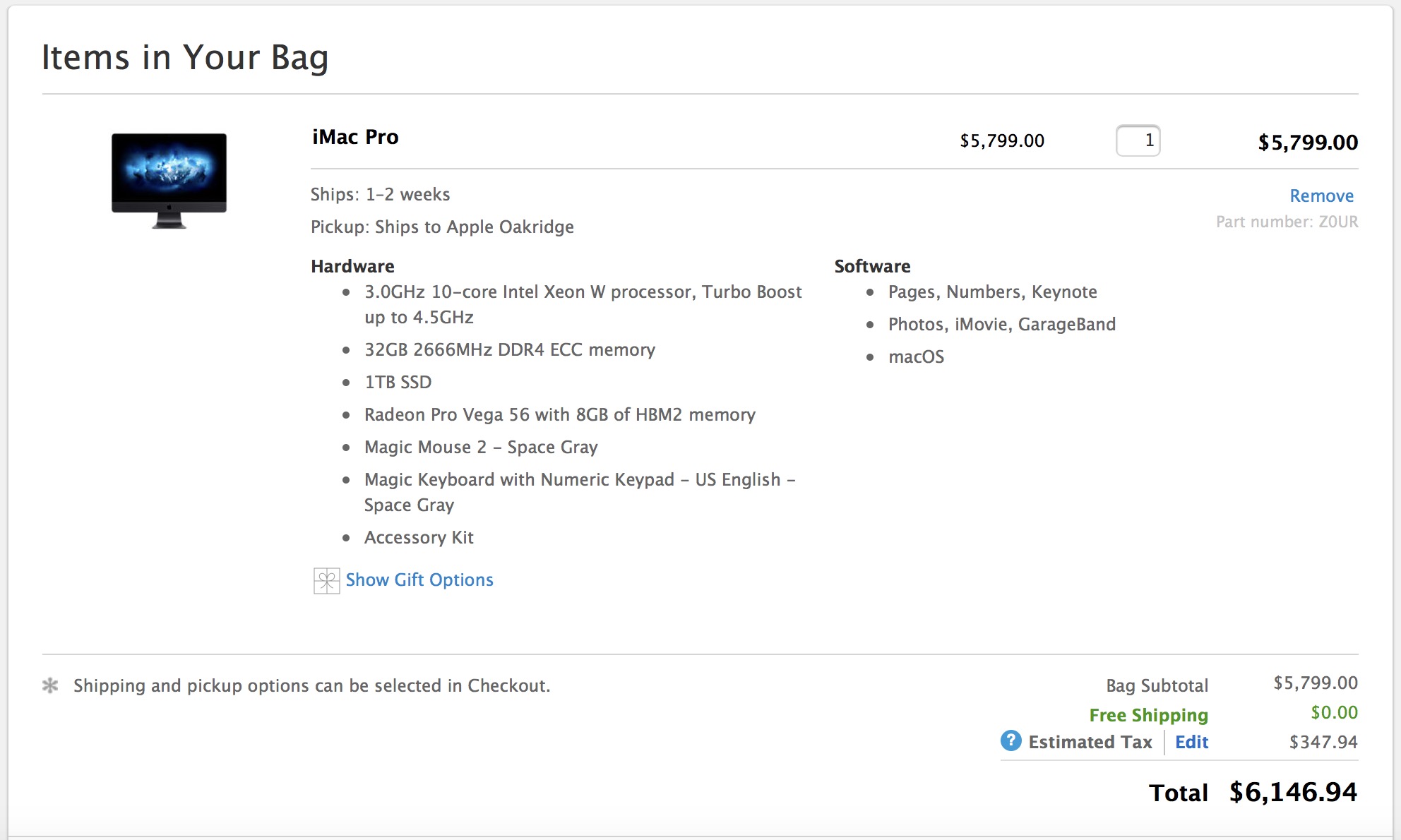This screenshot, framed by a narrow gray border against a white background, displays a detailed summary of an iMac Pro purchase. The screenshot is rectangular and oriented horizontally. In the upper left corner, the phrase "Items in Your Bag" is prominently displayed in black text. Below this heading, on the lower left, "iMac Pro" appears in bold black text, alongside a photo of the sleek black monitor.

To the right of the photo, the price is listed as $5,799, with a quantity of one unit specified. Further down, the expected shipping timeframe is noted as "Ships: 1-2 weeks," with the pickup location designated as "Apple Oak Ridge," both rendered in a lighter gray text.

Immediately beneath this is a section titled "Hardware" in bold black text. This section lists the hardware specifications in bullet points, including an accessory kit, a Magic Mouse 2, an ITB SSD, and 32 gigabytes of RAM.

Positioned in the upper right, the "Software" section, also in bold black text, outlines the pre-installed applications via bullet points. These include Pages, Numbers, Keynote, Photos, iMovie, GarageBand, and Macros. 

This comprehensive screenshot offers a clear and detailed overview of the iMac Pro purchase, including hardware specs, software applications, pricing, and availability.